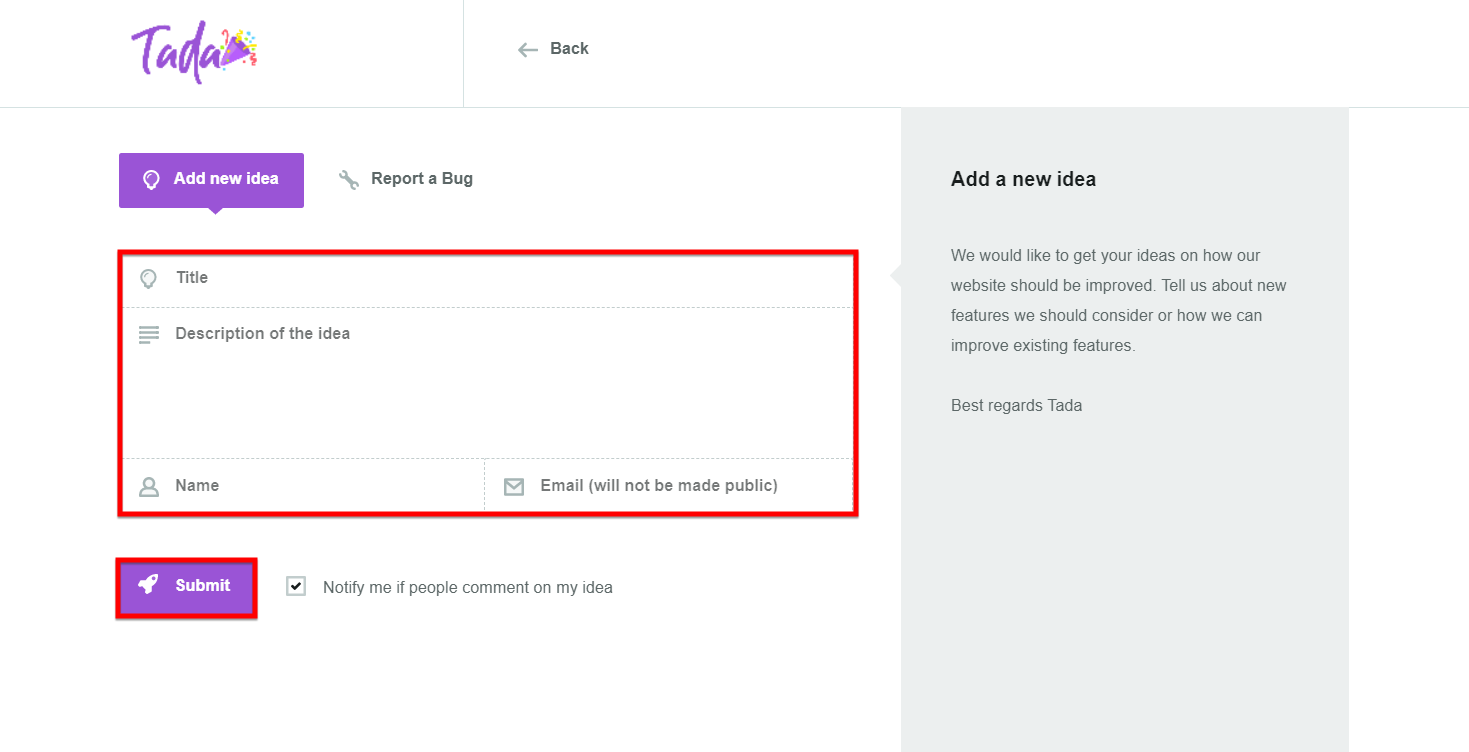The image captures a screen from the Tadah website, showcasing its logo and branding in the upper left corner, featuring a purple color scheme and a whimsical party popper hat at the end of the name. Adjacent to the logo, in the upper navigation panel, there is a back button for returning to the previous screen. The current screen is a user-friendly interface designed for customers to suggest new ideas. 

At the top of the main section, there is an "Add New Idea" button. Below this, users can find input fields to specify the title and description of their new idea, along with their name and email address (not publicly displayed). A "Submit" button is provided to finalize the suggestion. 

Additionally, there is an option to check or uncheck a box labeled "Notify me if people comment on my ideas," allowing users to opt-in or out of receiving feedback notifications. The page also includes a "Report a Bug" option, enabling users to switch from suggesting ideas to reporting issues they have encountered.

On the far right, a grey panel elaborates on the purpose of the screen, stating, "Add a New Idea: We would like to get your ideas on how our website should be improved."